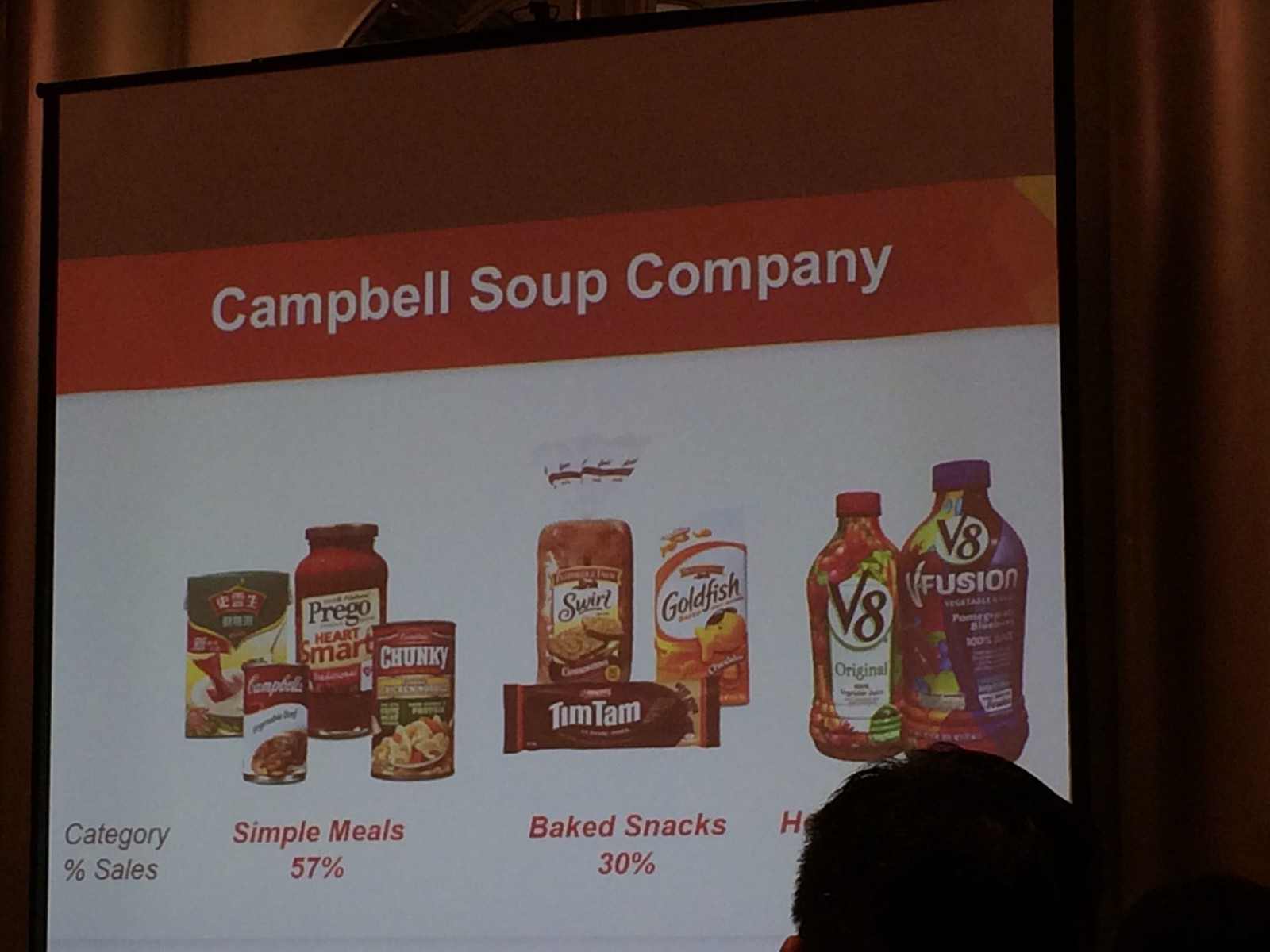This image captures a projection screen inside a ballroom, presumably during a corporate presentation or conference. The screen prominently displays information regarding the Campbell's Soup Company, set against a red and white background. The content on the screen is focused on "category percent sales," illustrated with various clusters of products. 

**Detailed Breakdown of the Image:**
- **Product Categories and Percentages:**
  - **Simple Meals:** Occupying the left portion of the screen, this category makes up 57% of sales. It includes images of soups and sauces.
  - **Baked Snacks:** This segment constitutes 30% of sales and features items such as bread and Goldfish crackers.
  - **Additional Products:** Some V8 bottles are also depicted, though specific details are obscured.

- **Shadow:** A shadow of a man's head is visible on the screen, indicating he is likely standing between the projector and screen, adding a sense of scale and context to the setting.

This detailed caption enhances the understanding of the scene, providing context about the location, content of the presentation, and the visual elements included in the photograph.